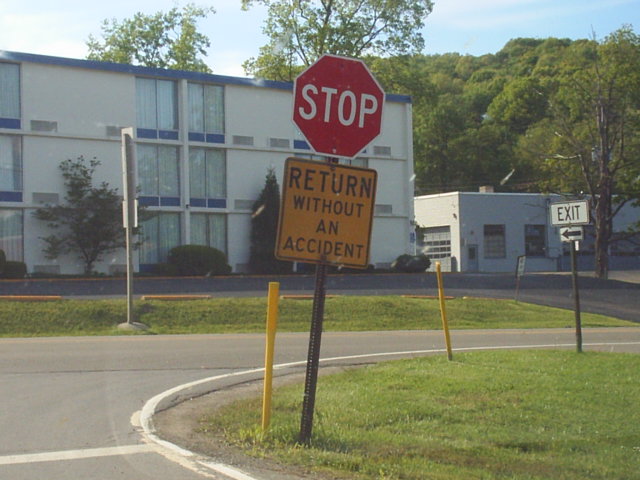In this real-life image, a metal pole stands at the corner of a road where it curves to the right. Attached to the pole are two distinct street signs: the lower sign is a yellow square with a black border reading "Return Without An Accident," while the upper sign is a red hexagon bordered in white with the word "STOP" prominently displayed in white letters in the center. To the left of this pole is a yellow post, approximately half the height of the street signs.

The scene is set on a small grassy section beside the road. Following the curve to the right, another yellow post is visible, and further along, a second metal pole with a white "EXIT" sign written in black letters can be seen. 

Across the road that intersects perpendicularly, a three-story white building with a blue border at the top is visible in the background. The building features large glass windows, and in front of it stands another street sign, seen from the back. To the right of this larger building is a smaller structure, beyond which a tree-covered mountain rises, adding a natural backdrop to the urban setting.